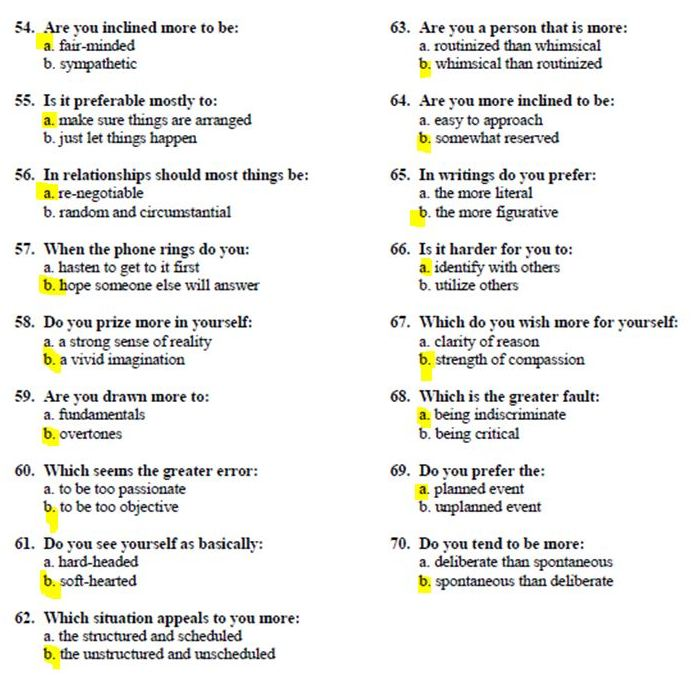The image depicts a detailed section of a personality quiz, featuring a series of multiple-choice questions printed in black text on a white background. Each question is paired with two options labeled A and B, with one option highlighted for each question, indicating the respondent's chosen answer. The questions are sequentially numbered, with the left column spanning from question 54 to 62 and the adjacent right column ranging from question 63 to 70.

Question 54, for instance, asks, "Are you inclined to be more fair-minded (A) or sympathetic (B)?" with the response "fair-minded (A)" highlighted. The questions cover various aspects of personality and decision-making preferences, such as:

- "In a relationship, most things should be negotiable (A) or random (B)?"
- "When the phone rings, do you feel the need to answer it immediately (A) or do you decide based on the situation (B)?"
- "Do you prize yourself more for a strong sense of reality (A) or vivid imagination (B)?"
- "Which seems the greater error: to be too passionate (A) or to be too objective (B)?"
- "In writing, do you prefer the more literal (A) or the more figurative (B)?"
- "Is it harder for you to identify with others’ feelings (A) or to utilize others (B)?"
- "Do you prefer planned events (A) or unplanned events (B)?"

These questions aim to reveal different facets of the respondent's personality by analyzing their preferences and tendencies in various scenarios.